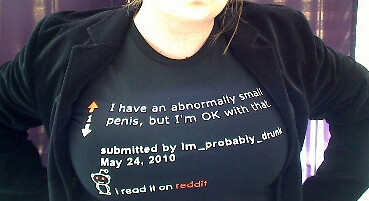This photograph features a woman dressed in a black jacket layered over a black shirt. The shirt prominently displays some text and graphics in white and orange fonts. Her neck and part of her chin are visible. The shirt's design includes an orange upward-facing arrow and a white number one. The white text states, "I have an abnormally small penis, but I'm okay with that." Below this message, "Submitted by I'm Probably Drunk, May 24, 2010" is also displayed in white font. Additionally, there is a small Reddit robot icon, incorporating white and orange colors, with the text "I read it on Reddit" shown, where "Reddit" is in an orangey hue. The image quality is clear, and there are no other visible elements or text on the shirt aside from these described details.